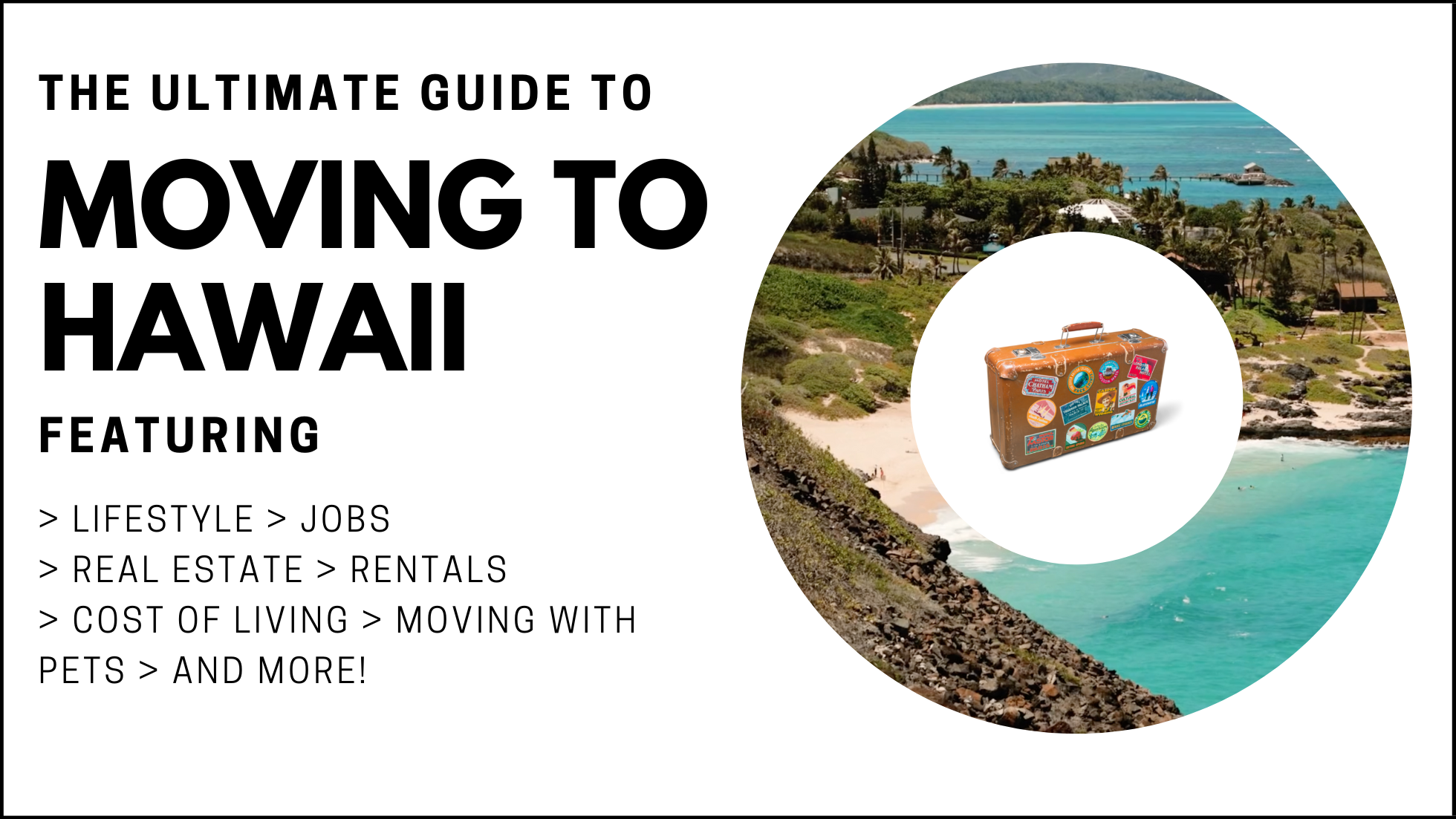This detailed image advertisement invites people to discover "The Ultimate Guide to Moving to Hawaii." Displayed on a clean white background, the left side features prominent black text detailing everything the guide includes: lifestyle, jobs, real estate, rentals, cost of living, moving with pets, and more. On the right side, a large circular photograph captures the essence of Hawaii with vivid blue waters, sandy beaches, lush green grasses, and tall palm trees, along with beachside cottages and huts. Nestled within this scenic larger circle is a smaller white circle containing an old-fashioned brown leather suitcase adorned with various travel stickers, symbolizing a well-traveled journey. The harmonious blend of natural beauty and practical information makes this advertisement both visually appealing and informative, perfect for anyone considering a move to the tropical paradise.